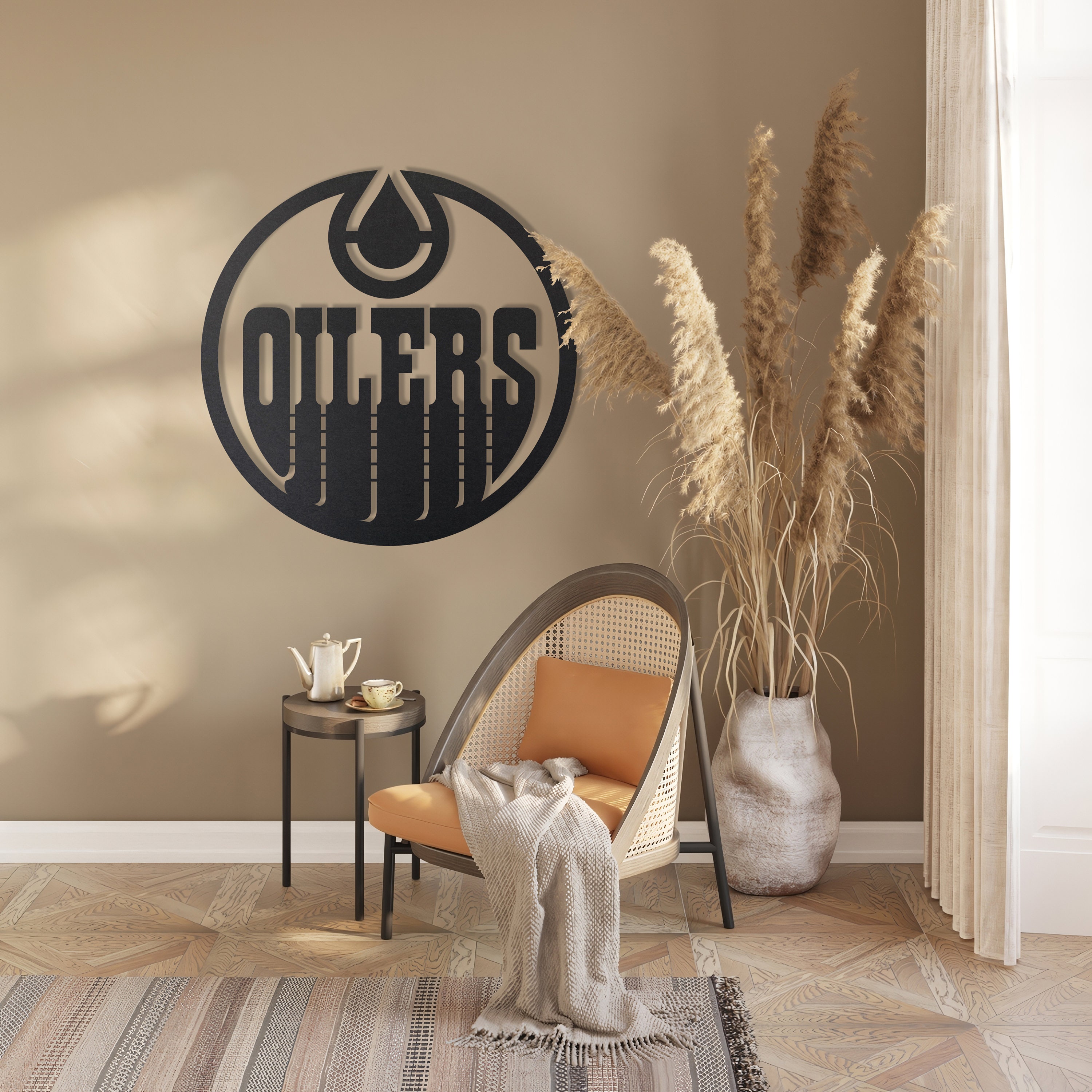This high-resolution, square-format photograph captures a professionally styled interior corner of a room with a meticulously arranged scene. In the foreground, a modern, rounded-back wicker chair with a dark-colored top and legs commands attention. The chair, featuring a distinct rattan design with holes, is adorned with two tan cushions and draped with a beige or white blanket. This chair is positioned partially on a patterned carpeted floor and a neutral-toned striped rug.

To the right of the chair, a large white stone-like pot houses decorative, feather-like plant plumes. Adjacent to the chair, on the left, stands a small side table holding a teapot and a tea cup with a saucer. The backdrop includes a tan wall decorated with a prominent wall hanging, bearing the word "OILERS" in black letters. This wall hanging is circular, with the bottom of the letters artistically bleeding into the lower part of the circle, evoking a modern and stylish look that complements the room's overall aesthetic. Curtains on the far right side extend from ceiling to floor, framing the scene with a touch of elegance.